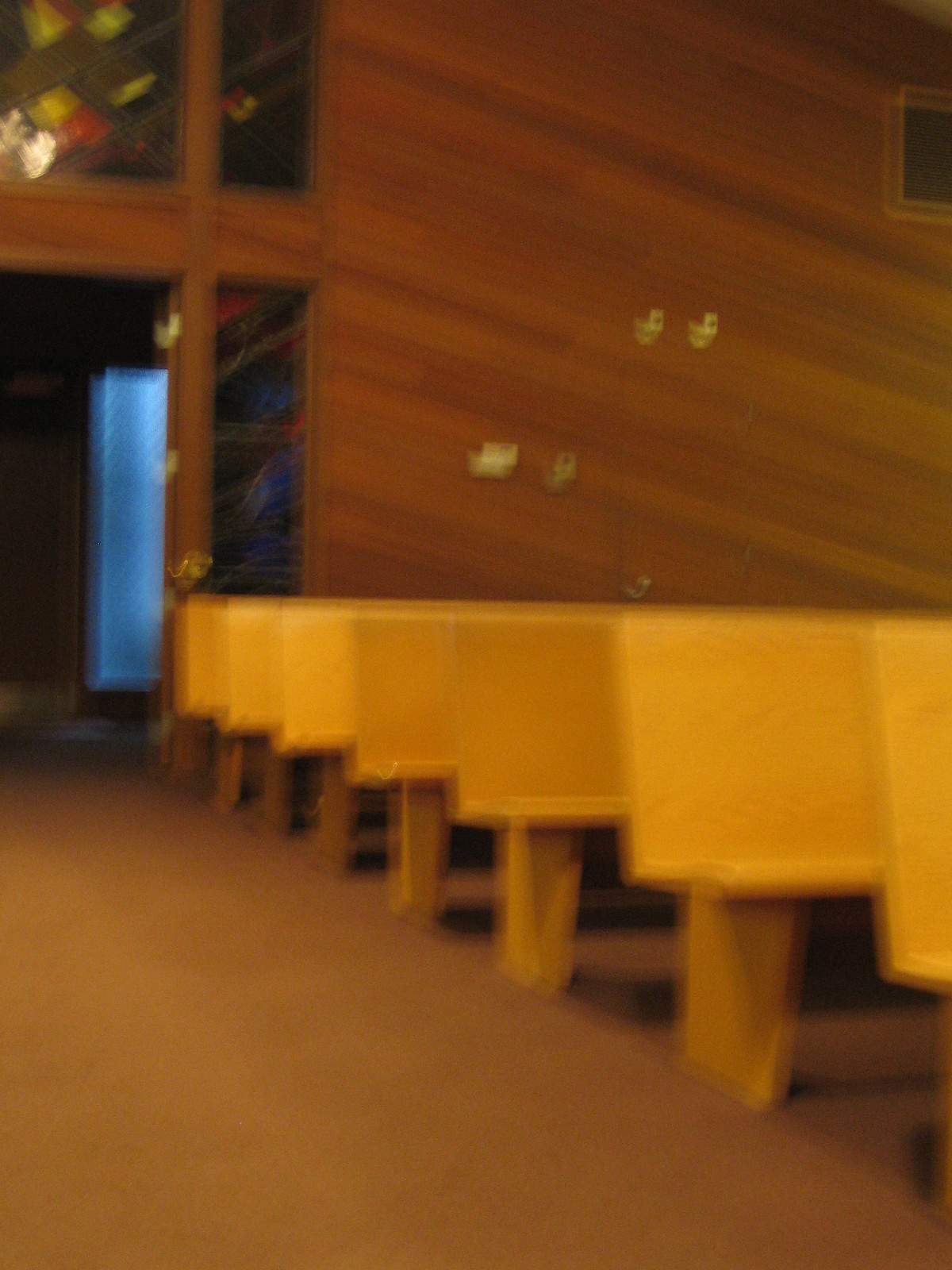This blurry color photograph depicts the interior of a place of worship, most likely a church. It captures the view from the central aisle, looking back towards the entrance. The image is poorly focused, obscuring finer details, but it reveals several key features. Six to seven rows of light brown wooden pews line the right side of the aisle, their exact texture indiscernible due to the blur. The floor appears to be a darker brown, and the back wall consists of white panels interspersed with rectangular windows. A large doorway at the back seems to lead to another area, featuring additional light coming through what could be a window or obscured by blue curtains. There also appears to be a color mural on one of the back walls. The overall atmosphere is indicative of a traditional church setting, illuminated by natural light filtering in through the out-of-focus windows.